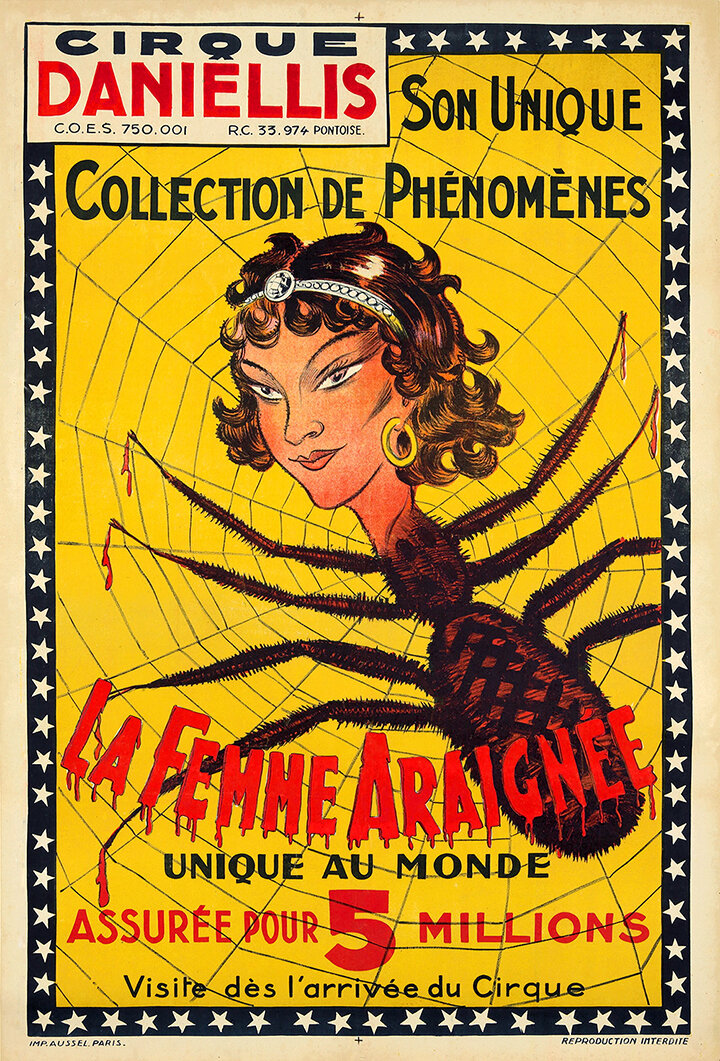This vintage poster, likely from an old circus or freak show, prominently features "Sir Danilis's Unique Collection of Phenomena." The main illustration is a striking and mysterious depiction of "La Femme Arachne," a creature with a spider's body and a woman's head. The woman, characterized by her curly red hair and adorned with a silver and gold headband featuring a black emblem, also wears gold earrings. The spider's legs stretch out dramatically within a web against a vibrant yellow background. Encircling the poster is a black and white banner embellished with stars and blood-dripping letters, adding to its eerie allure. The text includes phrases like "Unique Mondi" and "Assurée pour 5 millions," emphasizing the singular and extraordinary nature of the exhibit. The phrase "Cirque Dinellis" or "Cirque Danielus" in both Spanish and French, suggests this was an exhibition renowned for its unique and fascinating displays.